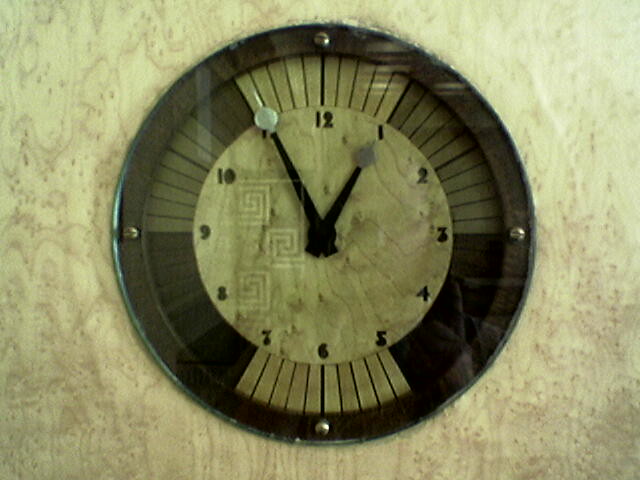The image features a sophisticated wall clock with a glass face mounted on a surface that appears to have a stone-like texture. The clock’s design is intricate, with a dominant glass surface in the foreground, secured by four visible screws positioned at the top, bottom, left, and right. 

The clock’s dial is composed of a series of concentric circles and radial lines. These lines extend almost to the outer black border, with some distinctions: the lines corresponding to the hour markers are bolder, while those marking each minute increment are finer. Additionally, every five-minute interval is marked by a noticeable change in shading. The shading gradient transitions from white to light gray, then to gray, and eventually to black, before starting the pattern anew.

The clock employs Arabic numerals for its hour markers, with '12' at the topmost position and '6' at the bottom. The hour and minute hands contrast each other in color: the hour hand is predominantly gray, while the minute hand appears white but is subtly shaded gray under the light. This meticulous design not only enhances readability but also adds a touch of elegance to the timepiece.